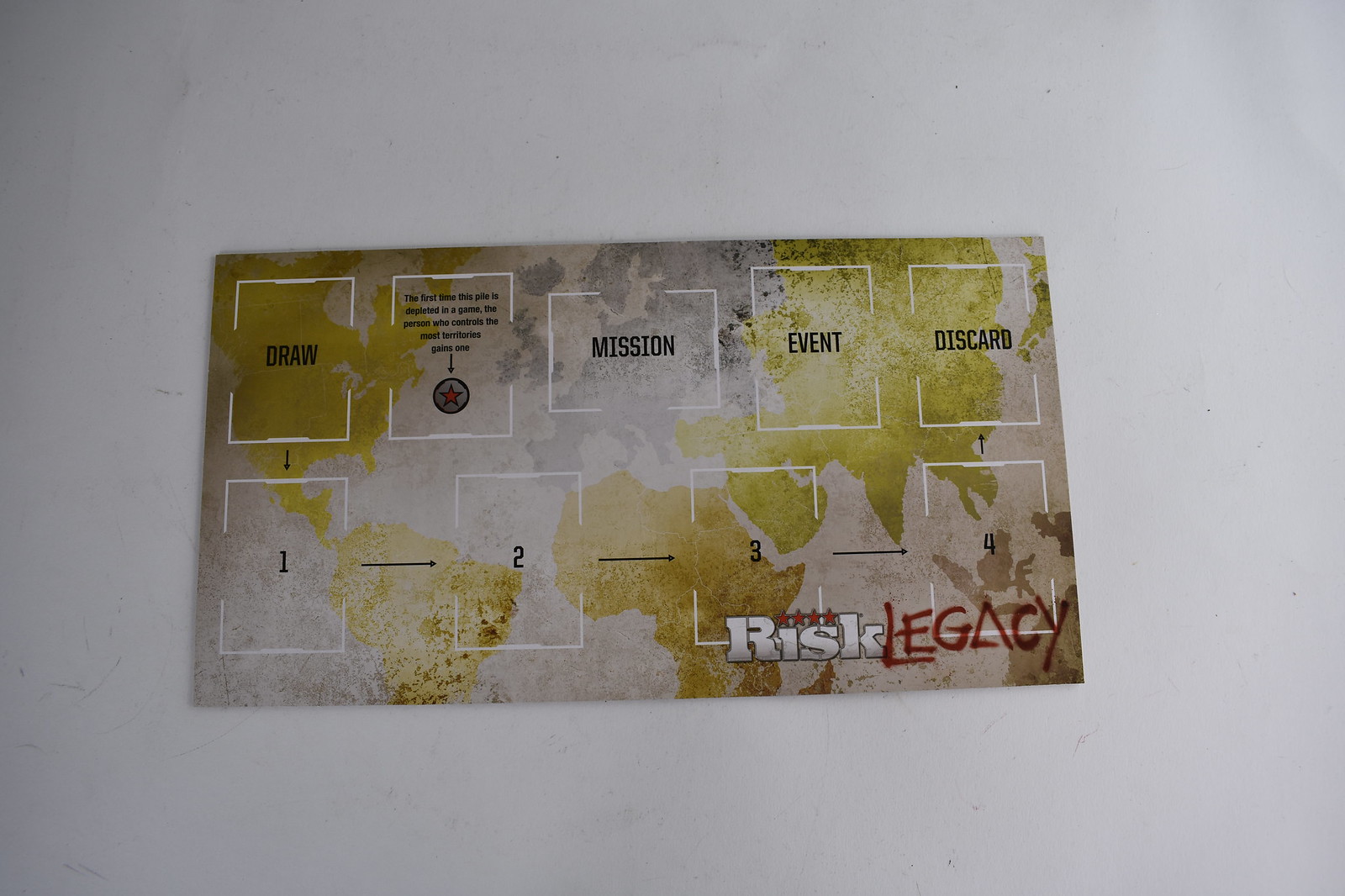The image shows a horizontally laid card, resembling a business card in shape, set against a plain off-white or light gray surface. The card, appearing to be an instructional component of the game Risk: Legacy, features a world map with continents colored in light green and Europe in light gray, over a soft gray ocean backdrop. Across the top, there are five labeled white boxes: "Draw," an unreadable second box with an arrow and a star, "Mission," "Event," and "Discard." Arrows connect these boxes in a sequence that begins at "Draw," moves down through numbered white boxes (1 through 4) at the bottom, and loops back up to "Discard." In the lower right-hand corner, the text "Risk Legacy" is prominently displayed, accompanied by four red stars, with "Legacy" written in a spray paint style font.